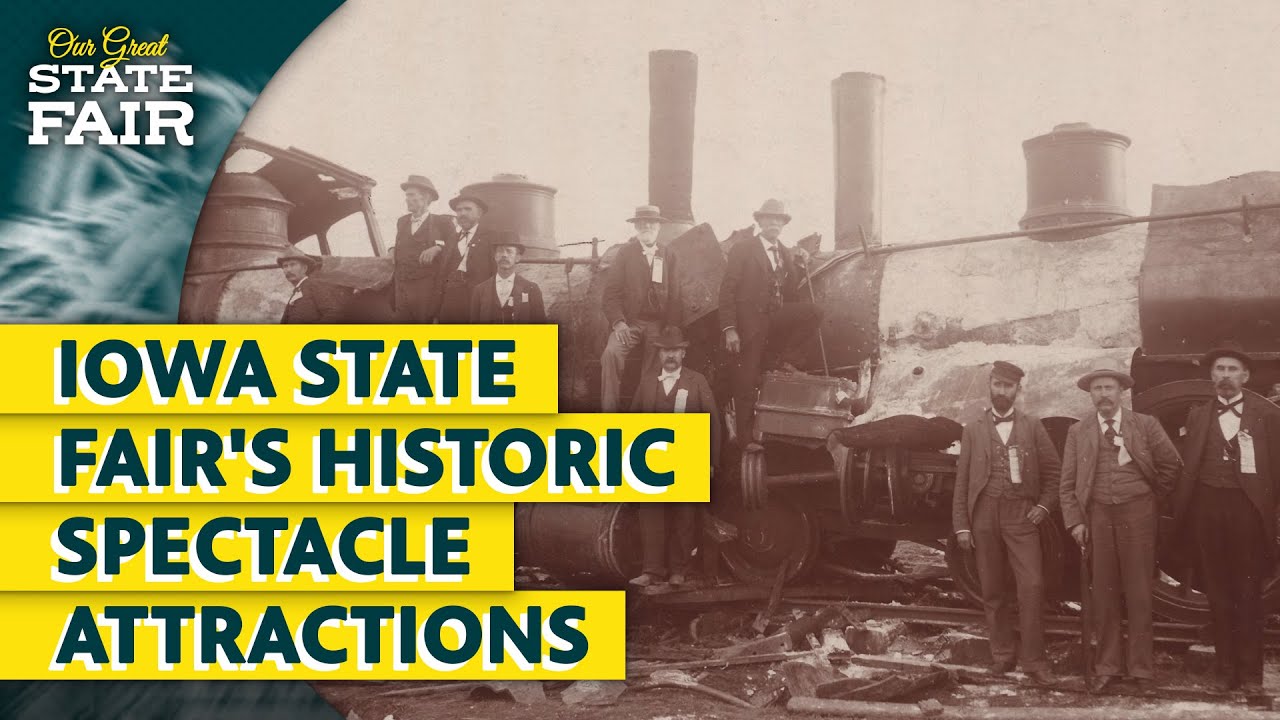The leaflet advertising the Iowa State Fair features a sepia-toned background image with a bronze and white hue. The scene captures an array of men congregated around what appears to be the aftermath of a locomotive crash. Scattered rusted metal fragments litter the foreground, with a prominent cylindrical piece—likely the front of an old locomotive—draped in silver metallic fabric on the left side of the image. 

In the bottom right corner, three men stand side by side, all dressed in light brown suits with white shirts. The man in the middle sports a long tie and a light-colored straw hat, while the two men flanking him don bow ties. The man on the far right wears a black top hat, and the man on the left has a black hat. Further in the background, a group of people can be seen climbing atop the wrecked locomotive, adding to the bucolic yet chaotic atmosphere.

To the left of the image, there is a verdant section with yellow cursive text reading "Are Great," immediately below which, in white block letters, is "State Fair." Towards the bottom left corner, four yellow bars, each inscribed with dark green letters with white shadows, read sequentially: "Iowa State," "Fairs Historic," "Spectacle," and "Attractions." These bars partially obscure some of the figures in the sepia-toned image.